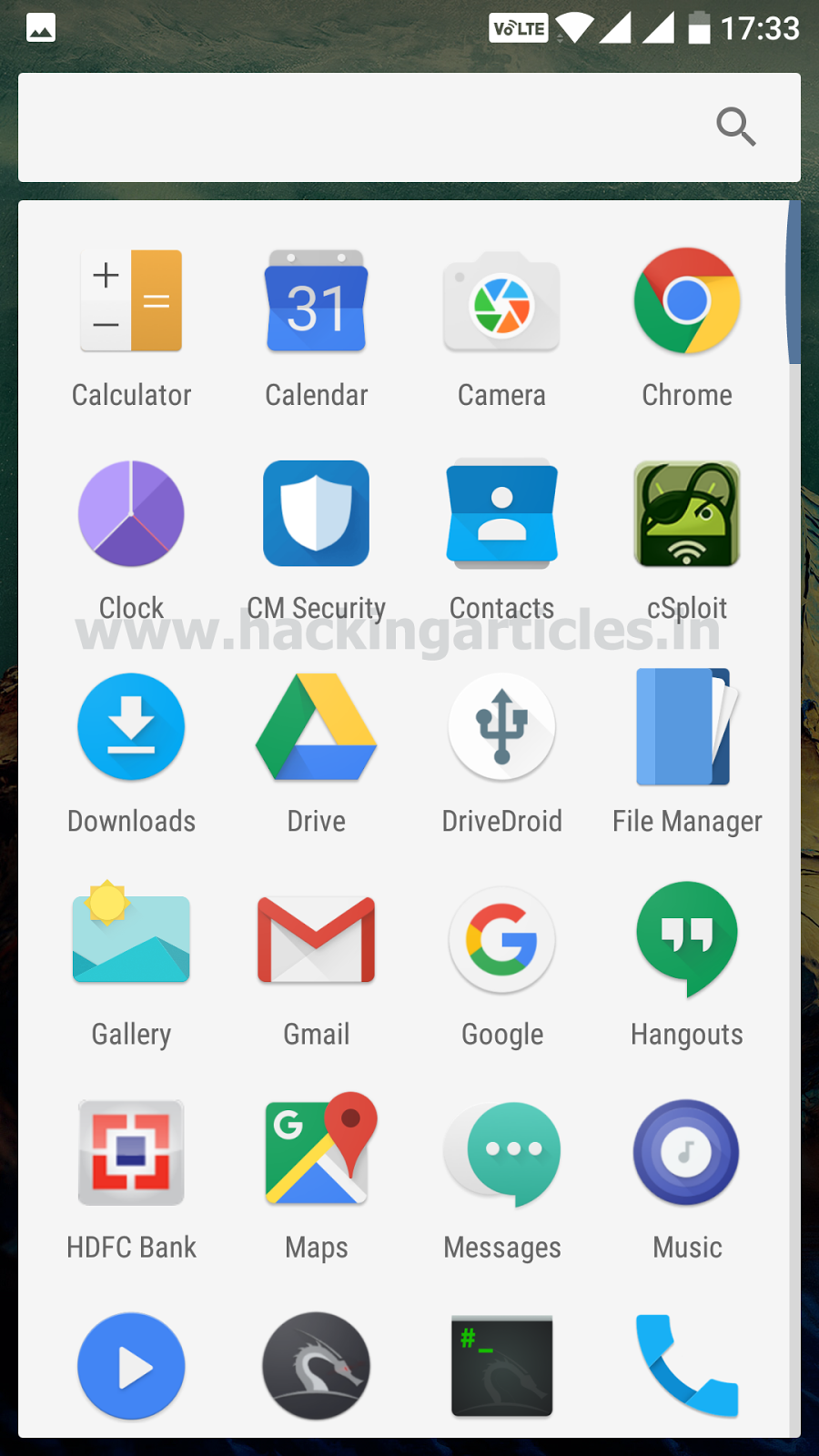In this image, we are looking at an app menu displayed on a smartphone screen, featuring a variety of icons arranged in a grid. Each icon is a square or circular symbol representing different applications:

1. The first icon features a distinctive half-and-half design with the left side in white and the right side in orange. On the white half, there are black symbols including a plus sign above a minus sign, while the right half contains a white equals sign.

2. The second icon resembles a calendar page with a page-flipping effect. It has a blue top portion that appears to be flipping down and displays the number "31". The background is gray with two small holes at the top, mimicking a physical page design.

3. The third icon is a camera with a lens comprising six triangular segments arranged in a circle, rotating clockwise. The colors of the triangles are dark blue, light blue, dark orange, orange, dark green, and light green.

4. The fourth icon is the recognizable Google Chrome logo, a circle with an inner blue circle surrounded by segments in red, yellow, and green, forming an outer ring.

5. The fifth icon is a clock face displaying three different shades of purple. The hands of the clock are white, set against a gradient purple background.

Following these detailed icons, other icons include apps such as CM Security, Contacts, C-Sploit, Downloads, Drive, Drive Droid, File Manager, Gallery, Gmail, Google, Hangouts, HCFC Bank, Maps, Messages, and Music, each represented by their standard icons.